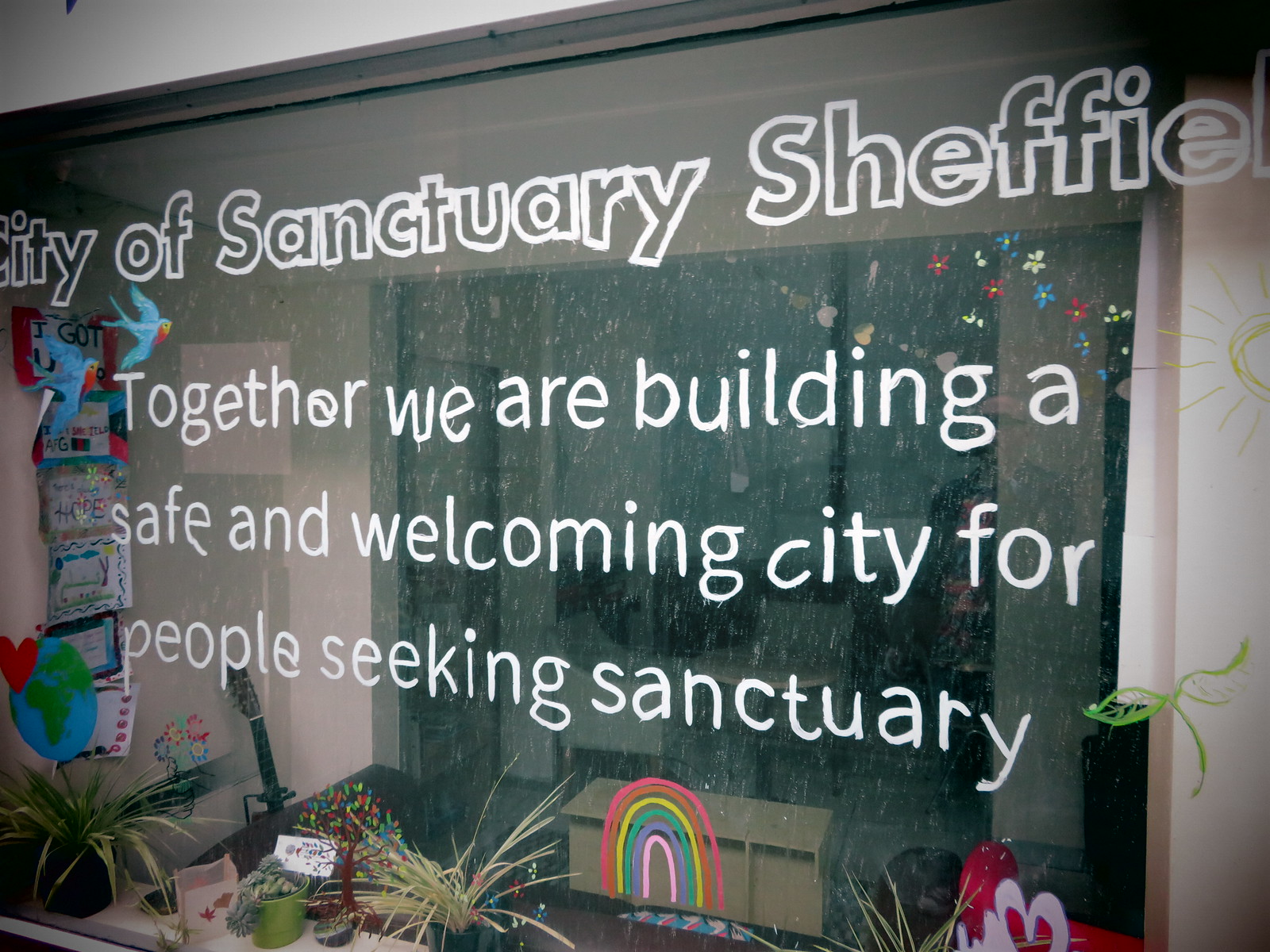This color photograph, in landscape orientation, captures the detailed view of a glass window on a City of Sanctuary Sheffield building. The window features a bold, black outline at the top and is framed by a beige stucco wall. Painted blue birds are seen flying on the top left corner, while a green and blue globe with a red heart is situated at the bottom left. The window displays white text that reads, "City of Sanctuary Sheffield" and beneath it, "Together, we are building a safe and welcoming city for people seeking sanctuary."

The glass is notably dirty with spots, adding a textured appearance. Through the window, an intriguing display is visible, albeit vaguely due to the dirt and low interior light. Inside, there are colorful items including a red heart, various plants, planters, and a guitar on the left-hand side. A green coffee cup sits on a shelf upfront, and a red and white design features prominently on the lower part of the window, depicting a white heart with something red behind it, a little green leaf at the top, and a yellow sun. A mailbox adorned with a rainbow motif is centrally placed at the bottom, enhancing the welcoming theme of the sanctuary.